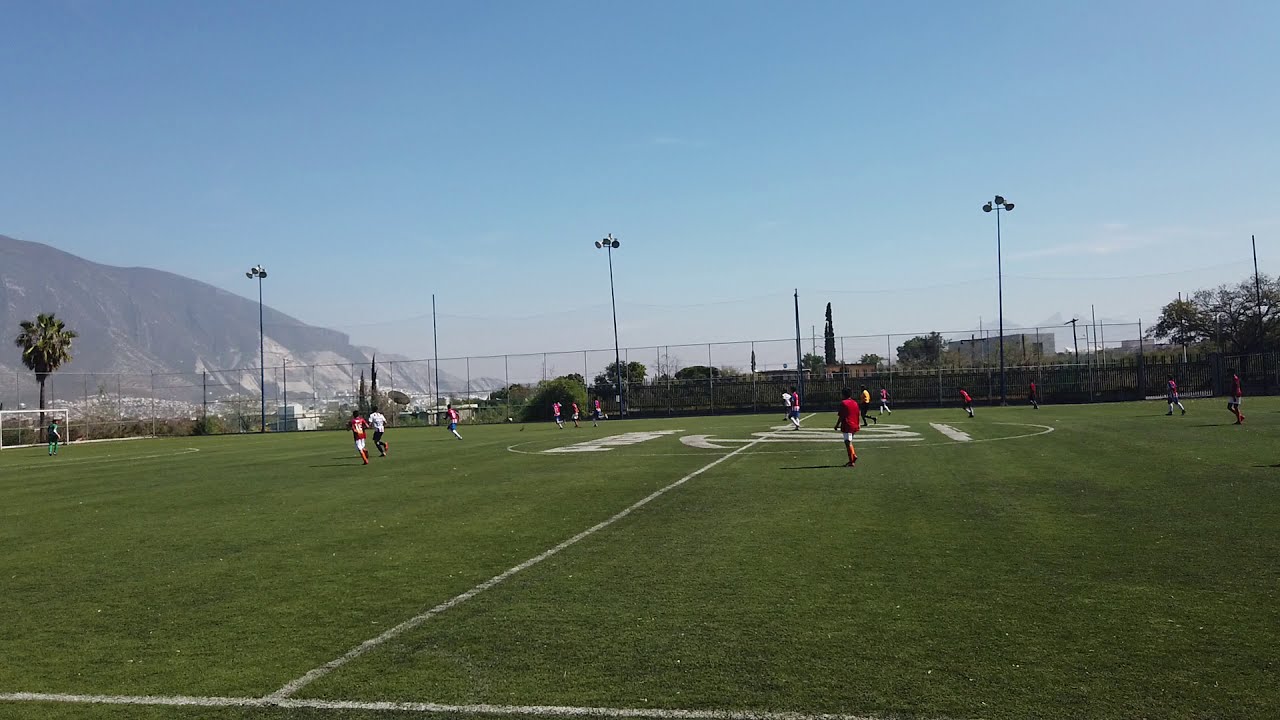In a vibrant color photograph of a soccer field, two teams, one in red uniforms and the other in white, are actively engaged in a game. The scene is set during daytime with a clear blue sky and minimal clouds. The grassy field stretches across the frame with the viewer’s perspective from the sideline. To the left, a goalpost is visible, while the tall fence encircles the field. Behind the fence, there are scattered trees, including a palm tree on the left and a pine tree towards the middle, alongside other greenery. This natural backdrop is accentuated further by a majestic mountain that meets the skyline. Three tall stadium lights rise above the fence, providing illumination to the serene landscape. The players are dispersed across the field, with their dynamic movements adding life to the picturesque setting.